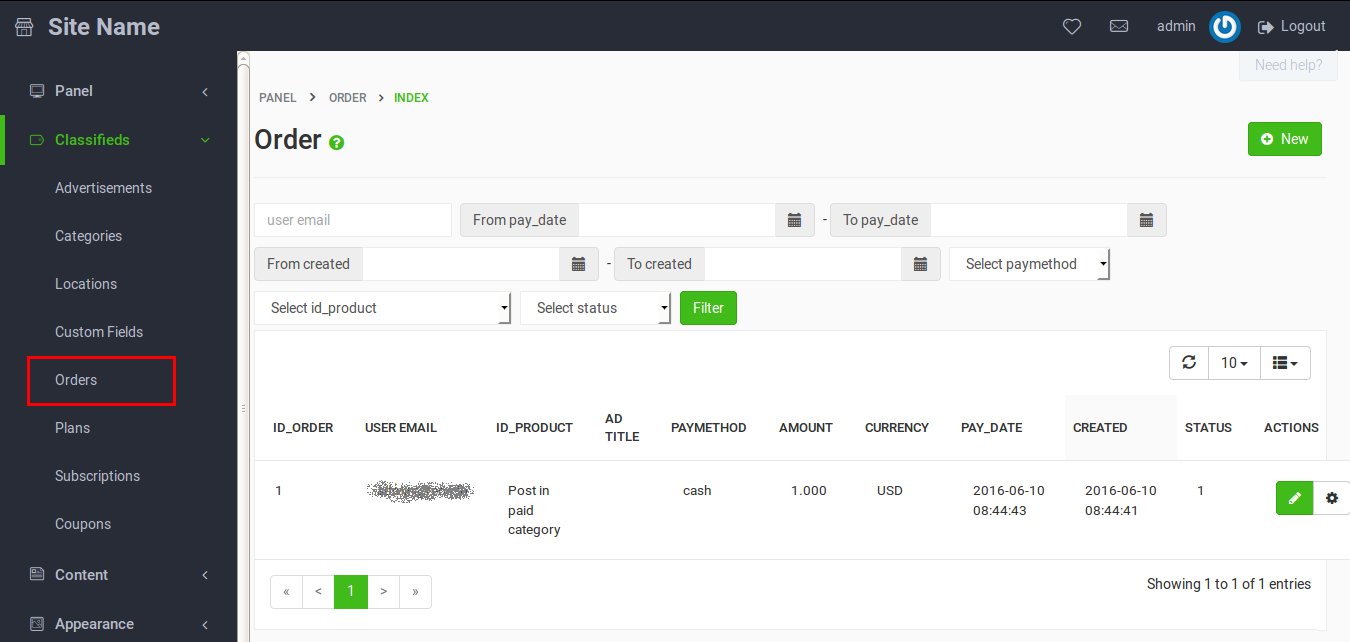This is a screenshot of a computer program used in a professional or company environment, likely for managing website orders. The interface is divided into several sections and features that are common in administrative tools.

At the very top left corner, the label "Site Name" is visible, suggesting that the user might be working on building a website or managing orders. On the right side of the header, there are icons for a heart, mail, admin features, and logging out.

The left sidebar includes a navigation menu with multiple options:
- **Panel**
- **Classifieds** (highlighted in green)
- **Advertisements**
- **Categories**
- **Locations**
- **Custom Fields**
- **Orders** (highlighted in a red rectangle, indicating the current active section)
- **Plans**
- **Subscriptions**
- **Coupons**

The main content area is currently displaying the "Orders" section, where the user needs to fill out fields for managing orders. The fields include user email, pay dates, creation date, current date, payment selection, product ID selection, and order status.

Below these input fields is a filter option, followed by a table with the following columns: ID order, user email, ID product, title, pay method, amount, currency, pay date, created, status, and actions.

An example order entry is displayed below, showing "Post in paid category", with the payment method listed as "Cash," amounting to one US dollar, and a payment date of June 10th, 2016.